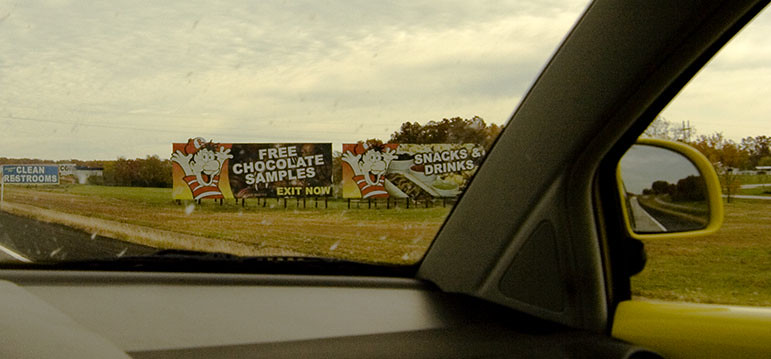The image offers a view from inside a vehicle, likely traveling along a highway, capturing a series of large billboards positioned on a grassy section by the roadside. In the background, the furthest billboard displays "Clean Restrooms" along with some smaller, unreadable text. Moving forward, two prominent billboards stand side by side on the ground.

The left billboard features a cheerful, human-like character wearing a red and white cap and shirt, with arms raised in excitement, announcing "Free Chocolate Samples - Exit Now." The right billboard shows the same character, equally enthusiastic, promoting "Snacks and Drinks," accompanied by images of various snacks and beverages. The text "and Drinks" is written in white.

Surrounding these billboards is a natural landscape with a cluster of trees that extend both in front of and behind the billboards, leading up to a picturesque lake encircled by additional trees in the distance.